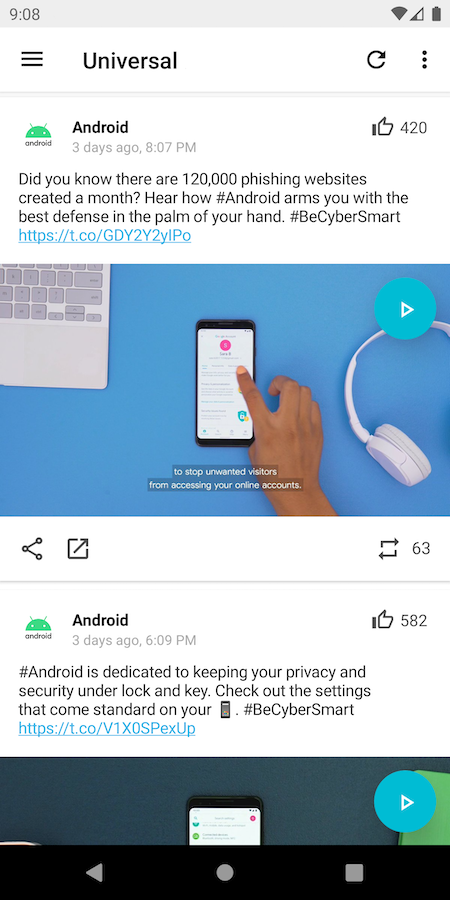A screenshot on a cell phone display shows various interface elements and a detailed social media post related to cybersecurity. At the top left corner, the time is displayed as 9:08, accompanied by icons indicating Wi-Fi signal strength, cellular signal strength, and a full battery. Below these icons are three horizontal lines stacked vertically on the left side, suggesting a menu or settings option, with the word "Universal" written next to them. On the right side of this section, a refresh button and a three-dot menu icon are present.

The main content of the screenshot features a post from an Android-themed social media account, published three days ago at either 7:07 or 8:07 PM. The post has garnered 420 likes. The message highlights cybersecurity awareness, stating, "Did you know there are a hundred and twenty thousand fishing websites created a month? Here at Android, we arm you with the best defense in the palm of your hand." The hashtags #Android and #BeCyberSmart follow the text, along with a shortened URL: https://t.co/gdy2y2yLpo.

In the image, a partial setup of a workspace is displayed, including a blue desk, a cell phone, and a keyboard, with someone’s hand interacting with the phone. The caption on the screen reads, "To stop unwanted visitors from accessing your online accounts."